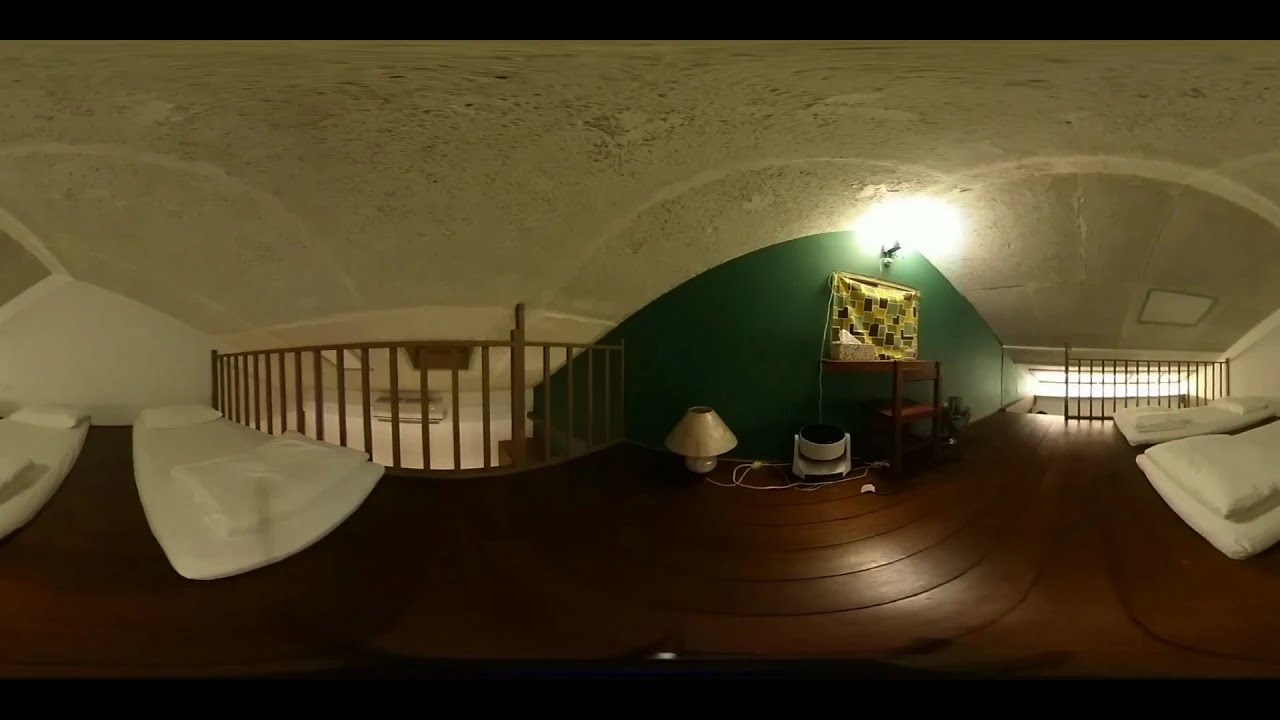This image captures a heavily distorted panoramic view of a loft area inside a home. The horizontally aligned rectangular picture, bordered in black at the top and bottom, reveals a variety of elements in this upstairs room. The loft is furnished with four floor mattresses, each equipped with a pillow and folded sheets at the foot of the bed. On the ground, there is a white lamp with its cord visible and what appears to be a humidifier beside it. A wooden railing runs along the edges of the loft, safeguarding the area and offering a glimpse down to the lower level. 

The floor is made up of dark brown wooden tiles with curved sections, adding a unique texture to the space. The green wall, located centrally in the image, is slightly curved and features a checkered curtain in green, black, and yellow, possibly covering a window or screen. Additionally, a small wooden desk sits beneath this colourful curtain, holding a box of tissues. The slanted ceiling, covered in a textured white or beige material, follows the shape of the roof, giving the room a cozy, enclosed feel. A staircase is situated next to the railings, indicating the loft's entrance point.